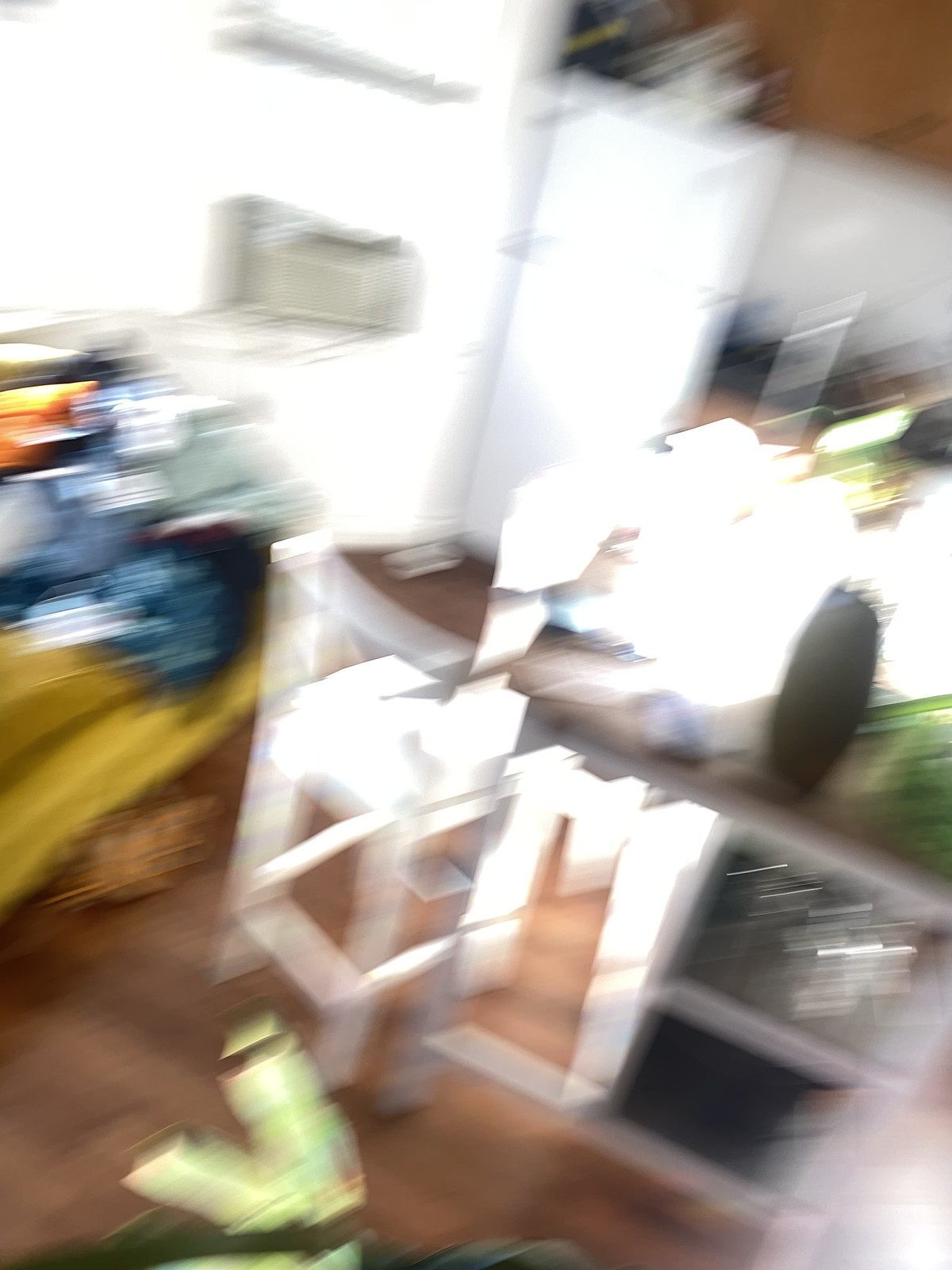This extremely blurry and distorted image appears to be taken indoors, possibly within a kitchen or laundry room. Dominating the center is a tall, white bar stool or chair, situated near what might be a countertop or table with a brown top. Behind the stool, there's a large white rectangular object which could be a refrigerator or a door. To the left of this, a white wall features a small gray box-like technology, potentially an air conditioner control. Below this, a pile of multi-colored items—possibly clothes or trash—rests on the floor. On the countertop behind the stool, various indistinguishable objects can be seen, amidst the light breaking in from a window. The overall scene is heavily blurred with significant glare, making finer details, like the exact nature of objects or the room's purpose, hard to discern. The floor appears to be wooden. Additionally, there are scattered green and yellow objects, and a potential futon with clothes on the left side of the image.